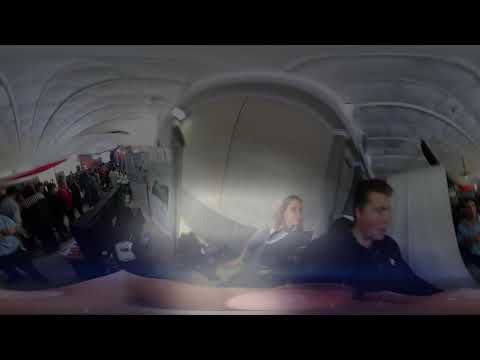The image showcases an interior setting, likely an office, airport, or ship, characterized by a 360 panoramic distortion that curves straight lines. Centered towards the bottom right, there's a Caucasian man with short hair in a blue shirt walking, accompanied by a woman with long, blondish hair and a blue and white shirt. The woman seems to look at him as they move towards the bottom right. To the center-left, a large crowd stands in line amid various colored outfits like red, black, white, and blue, suggesting an industrial or commercial environment. Beige walls, a tan desk, and a white metal ceiling form the backdrop. The image lacks text and has a blurry, faded quality with a flash of light over the center and the woman's face.